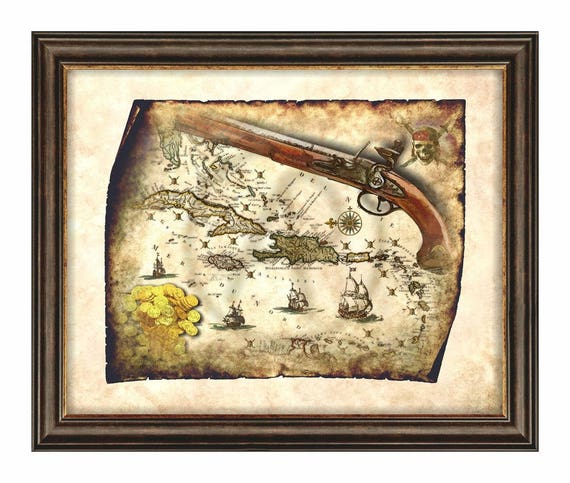This detailed artwork, framed in a rectangular wooden frame, depicts an old-timey pirate map rendered on weathered parchment. Dominating the top right corner of the map is an ominous skull and crossbones icon, symbolizing danger and piracy, just beneath which lies an old flintlock gun intricately painted into the map. A collection of Caribbean islands, surrounded by ships, serves as the central focus, with numerous skull and crossbones icons scattered across the waters, marking sites of piracy. In the bottom left corner, the map features gold coins and the aftermath of a cannonball explosion, further enhancing the pirate theme. The entire illustration is characterized by a yellow and green color palette, with crinkled and folded edges, enhancing its antiquated and adventurous aesthetic.